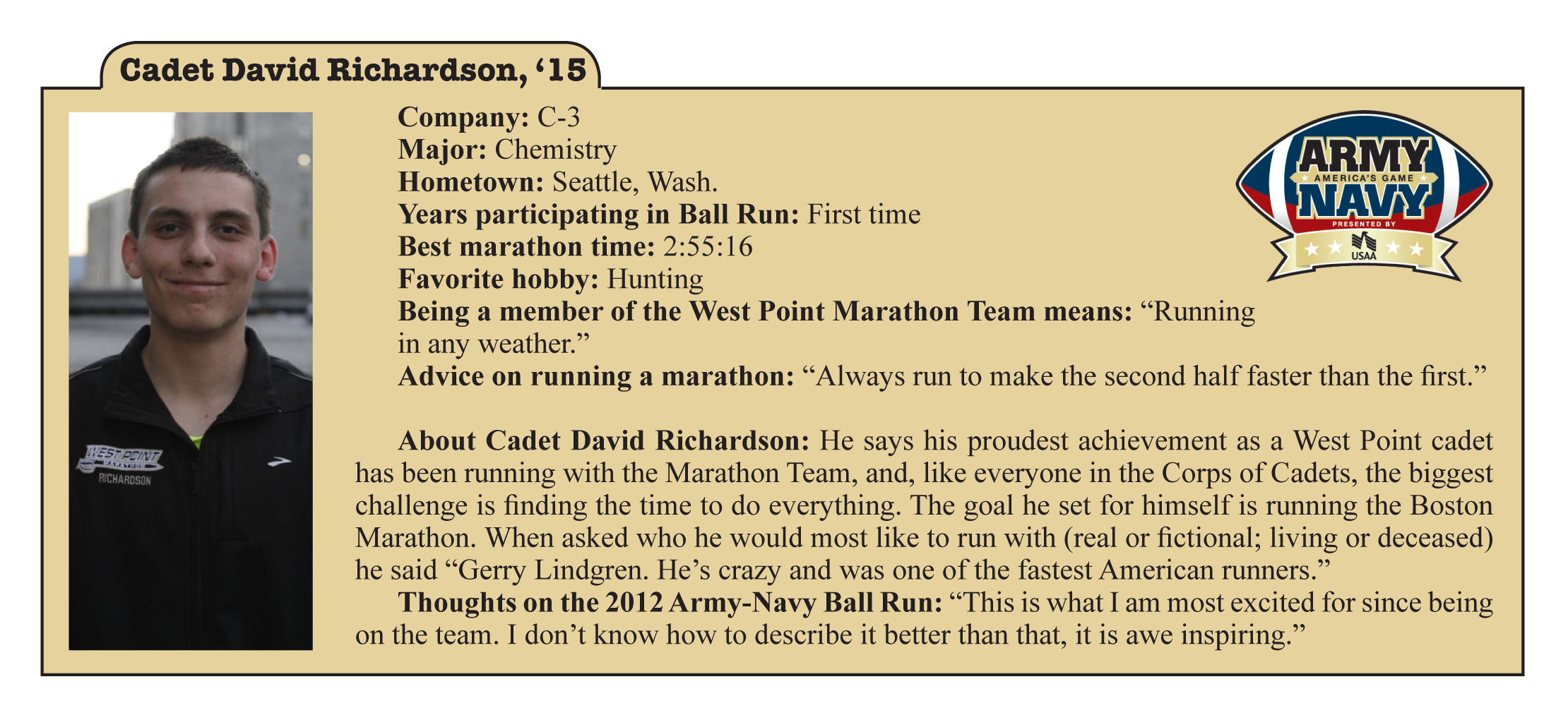This graphic resembles an old-school recipe card with a small tab marking the top left corner. The tab reads "Cadet David Richardson '15." The entire card has a light brown background and contains detailed information about Cadet Richardson, who is featured wearing a black polo shirt with a logo on it. His image, which shows him from the midriff up, occupies the left side of the card. He has short black hair and a closed-lip smile, standing in front of a backdrop that hints at a gray building under a white sky.

Positioned in the upper right corner, a football graphic with blue and red halves proudly states "Army, Navy, America's Game," underlined by a banner with four white stars and a bird symbol above the word "USAA." This indicates the card's association with the Army-Navy football game.

Directly below the tab with his name, several informational sections describe Cadet Richardson’s background and achievements:
- **Company:** C3  
- **Major:** Chemistry  
- **Hometown:** Seattle, Washington  
- **Years Participating in Ball Run:** First Time  
- **Best Marathon Time:** 2:55:16  
- **Favorite Hobby:** Hunting  

One highlighted quote captures his feelings about his hobby: "Being a member of the West Point Marathon Team means running in any weather." Additionally, a notable personal goal mentioned by Cadet Richardson is to run the Boston Marathon. His pride in his achievements is expressed through quotes and a reflection on his experiences: "This is what I am most excited for since being on the team. I don't know how to describe it better than that. It is awe-inspiring."

An inspirational quote about running is also included: "Always run to make the second half faster than the first," enhancing the motivational tone of the card. Cadet Richardson’s admiration for Jerry Lindgren, one of America's fastest runners, further emphasizes his dedication and passion for running.

In summary, this detailed card serves as both a biographical insight and a tribute to Cadet David Richardson, encapsulating his academic, athletic, and personal achievements alongside his aspirations and motivations.